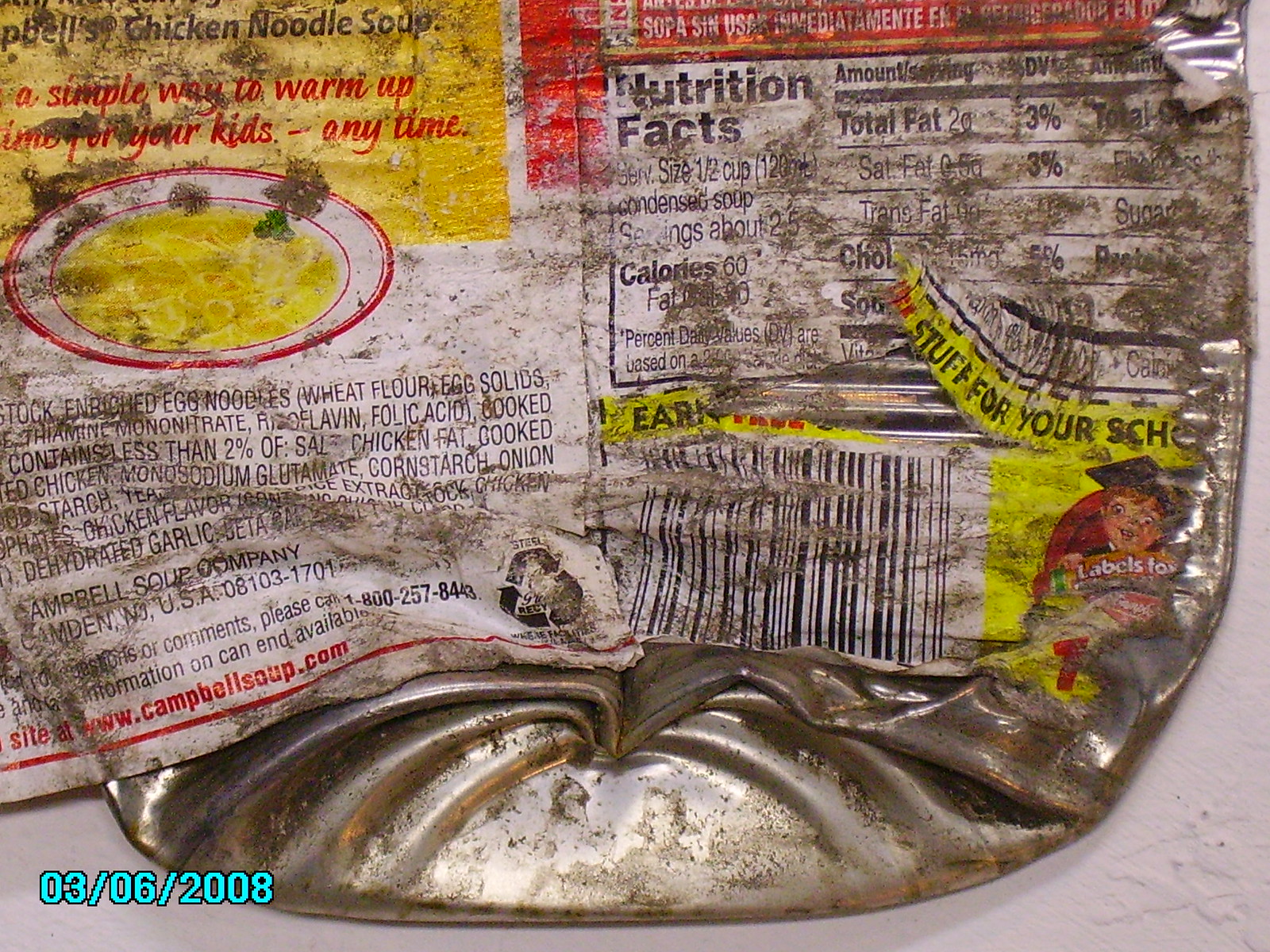This photograph, captured in close-up on March 6, 2008, displays the bottom portion of a heavily crushed and mangled Campbell's Chicken Noodle Soup can. The can's condition is notable for extensive creasing and visible dirt, with spots of rust on its lower section. Highlighting catches the light on the right and bottom sides of the can. The label, a mix of white, black, red, yellow, and silver-gray tones, includes nutritional information on the right and ingredients on the left. The upper-left corner of the label identifies it as Chicken Noodle Soup, accompanied by an illustration of a bowl containing ring noodles in broth. The image is framed with a light blue date stamp in the lower left corner, bordered in black.